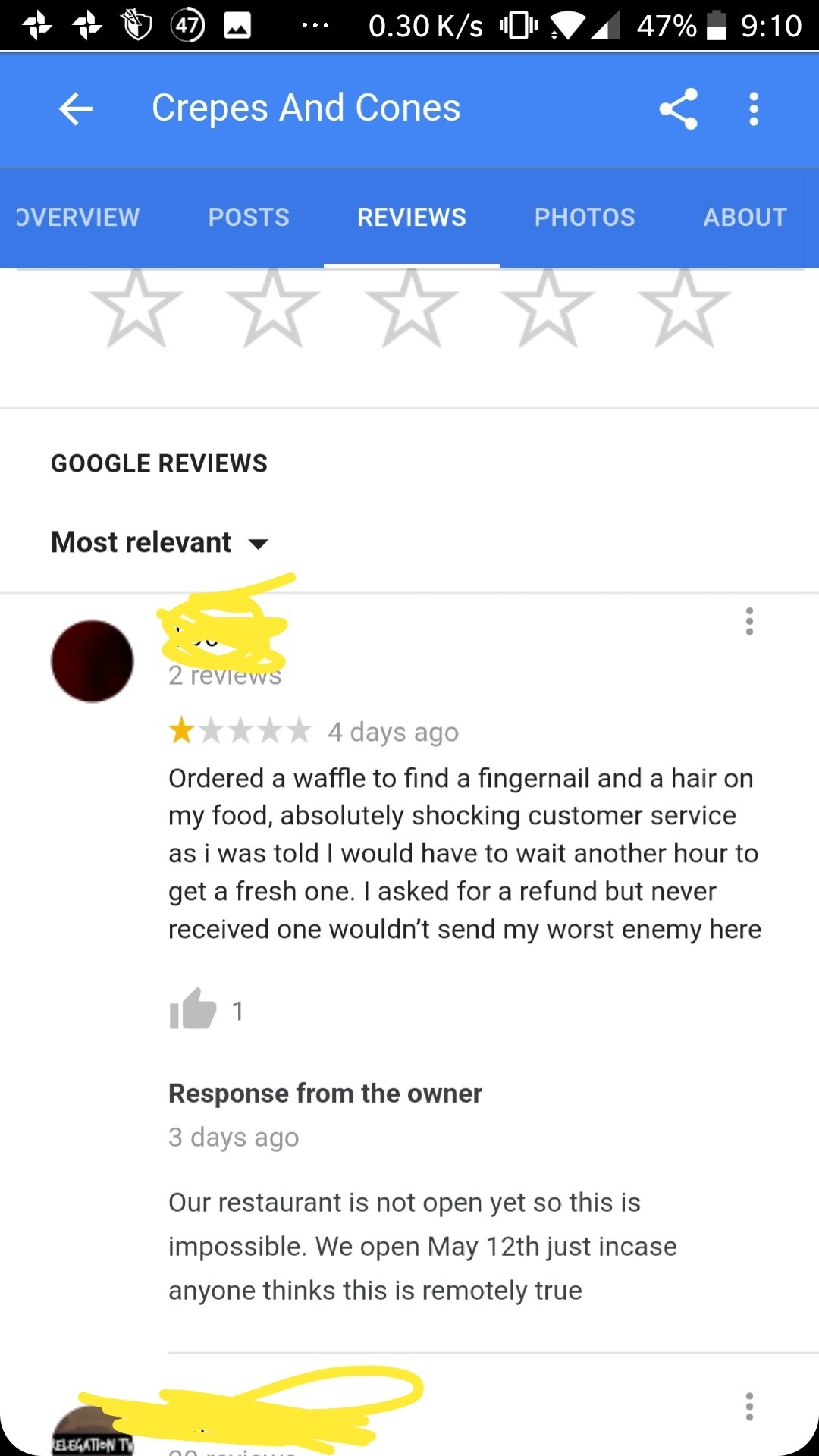**Caption:**

Screenshot of an online review for "Grapes and Cones" restaurant, depicting a one-star rating. The review describes an appalling experience where the customer found a fingernail and hair in their waffle, alongside poor customer service that required an hour's wait for a replacement and a refund that was never provided. The reviewer concludes by stating they wouldn't recommend the restaurant even to their worst enemy. Beneath this review, a response from the owner refutes the allegations, clarifying that the restaurant hasn't opened yet and is scheduled to open on May 12th, suggesting the review is fabricated. The original review was posted four days ago, with the owner's rebuttal appearing three days ago.